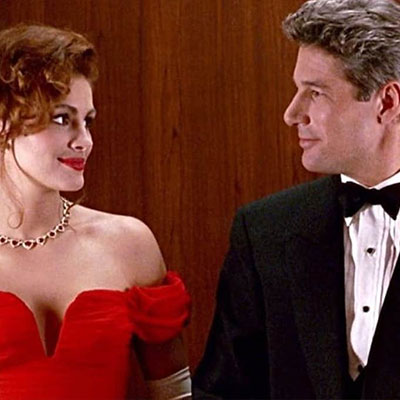This image is a screenshot from the movie Pretty Woman, featuring Julia Roberts and Richard Gere standing against a rich, dark cherry wood background. Julia Roberts, a white woman with fiery red hair styled up and curly, is seen on the left wearing a stunning strapless red dress that hangs off her shoulders. She complements her elegant attire with long white gloves that reach just above her elbows, a gold necklace adorned with hearts, and striking red lipstick. Julia is gazing lovingly at Richard Gere with a smile on her face. Gere, a white man with brownish-gray hair, is dressed impeccably in a black tuxedo paired with a white shirt that has black buttons down the front and a black bow tie. He looks back at Julia with a tender expression, capturing a romantic moment as they stare into each other's eyes.